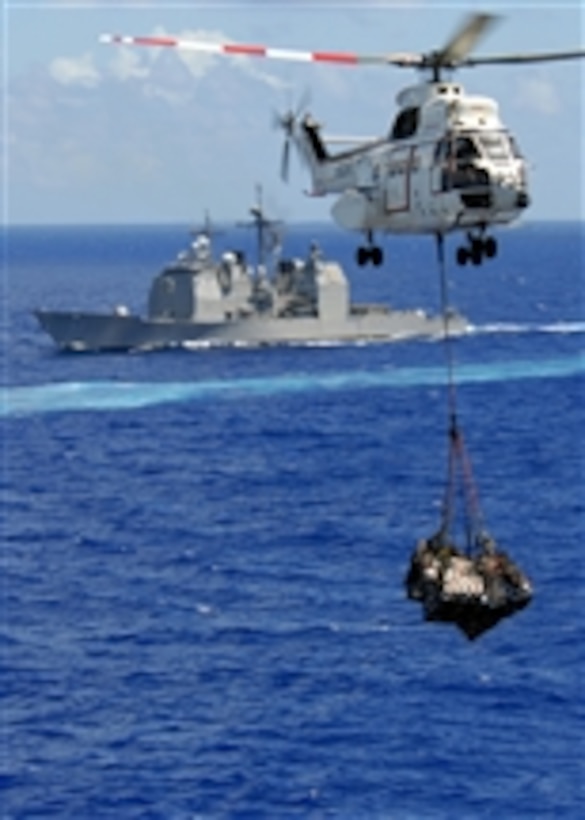In this color photograph, a white helicopter with a distinctive red and white top propeller and a black tail propeller hovers in the foreground, showing clear flight dynamics with wheels down and a long rope dangling beneath it. Attached to the rope is a net, containing a blurry, indeterminate circular object. Below the helicopter, dark blue choppy waters spread across the majority of the image, giving off nuanced hues with a lighter blue section just in front of a boat. In the background, a gray-silver destroyer-like military ship navigates these turbulent waters without any visible markings. Above, the sky is a serene light blue, adorned with wispy clouds, setting a stark contrast against the active scene below. The composition of the photograph places the helicopter prominently in the bottom right quadrant, while the ship lingers in the upper middle, painting a dynamic interrelation between air and sea operations.